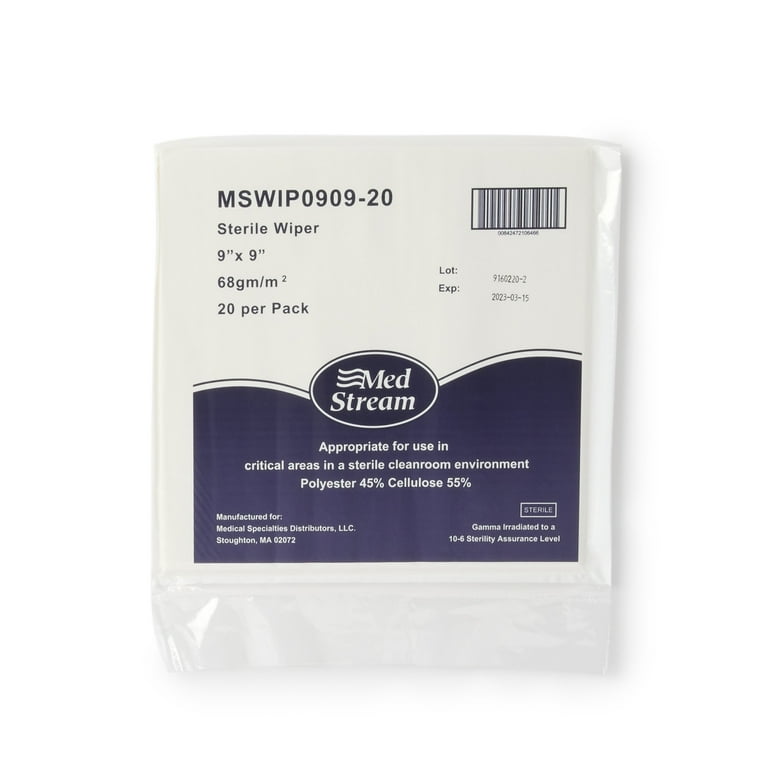The image features a close-up view of a square, white, plastic package containing sterile wipes. The top half of the package is primarily white, while the bottom half is a mild shade of violet. In the top left corner, black writing displays a product number, MSWIP0909-20, followed by the description: "sterile wiper, 9 inches by 9 inches, 68gm/m2, 20 per pack." Below this text is a large, violet-colored oval outlined in white, housing the brand name "Medstream"—with "MED" positioned above "STREAM" in white letters, accompanied by three wavy white lines. 

On the right-hand side of the package, a rectangular UPC barcode is situated next to the lot number and expiration date, although the dates are too small to be legible. Beneath the brand name, additional text in white reads: "appropriate for use in critical areas in a sterile cleanroom environment, polyester 45%, cellulose 55%". The bottom left corner contains the manufacturer's information, while a small white rectangle in the bottom right corner, on a violet background, states "sterile". The object is centered within the image, with all text and features clearly visible.